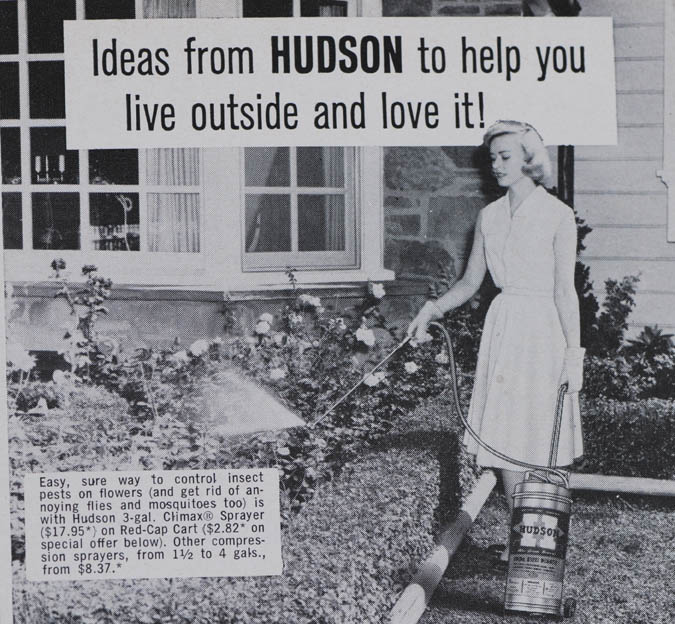This black-and-white photograph, likely from the 1950s or 1960s, captures a detailed advertisement for Hudson insect control products. A stylish woman stands in a manicured garden outside a stone house with large windows, wearing a white dress and gloves. Her short blonde hair is curled neatly, typical of the era. She is using a Hudson-branded canister sprayer with a hose and a long rod, misting her flower bed to control pests. The background text in a white rectangle at the top reads, “Ideas from HUDSON to help you live outside and love it!” emphasizing the brand. Another smaller white rectangle in the lower left corner provides additional details, stating: “Easy, sure way to control insect pests on flowers, and get rid of annoying flies and mosquitoes too, is with Hudson 3-gallon Climax Sprayer, $17.95 on Red Cap Cart $2.82 on special offer below. Other compression sprayers from 1.5 to 4 gallons, starting at $8.37.” The advertisement showcases both the product and its practical application in a domestic setting.